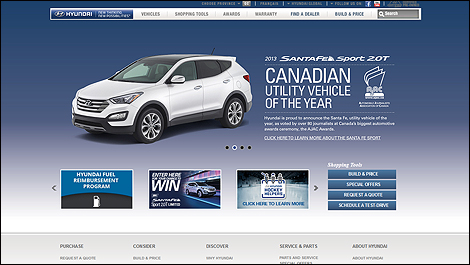Cropped screenshot of the Hyundai homepage showcasing a sleek blue-themed design. At the top, a crisp white bar features the Hyundai logo on the left, followed by categories such as "Vehicles," "Shopping Tools," "Airbags," "Warranty," "Find a Dealer," "Build and Price," and a search button to the far right. Dominating the body of the webpage, a Hyundai Santa Fe Sport sits angled against a blue backdrop, flanked by the text "Canadian Utility Vehicle of the Year" and accompanied by an image of an award and a descriptive paragraph underneath. At the bottom, a set of three thumbnails is navigated by arrows on each side, allowing for easy scrolling. Adjacent to the thumbnails, a small row of boxes under the heading "Shopping Tools" offers options like "Build and Price," "Special Offers," "Request a Quote," and "Schedule a Test Drive."